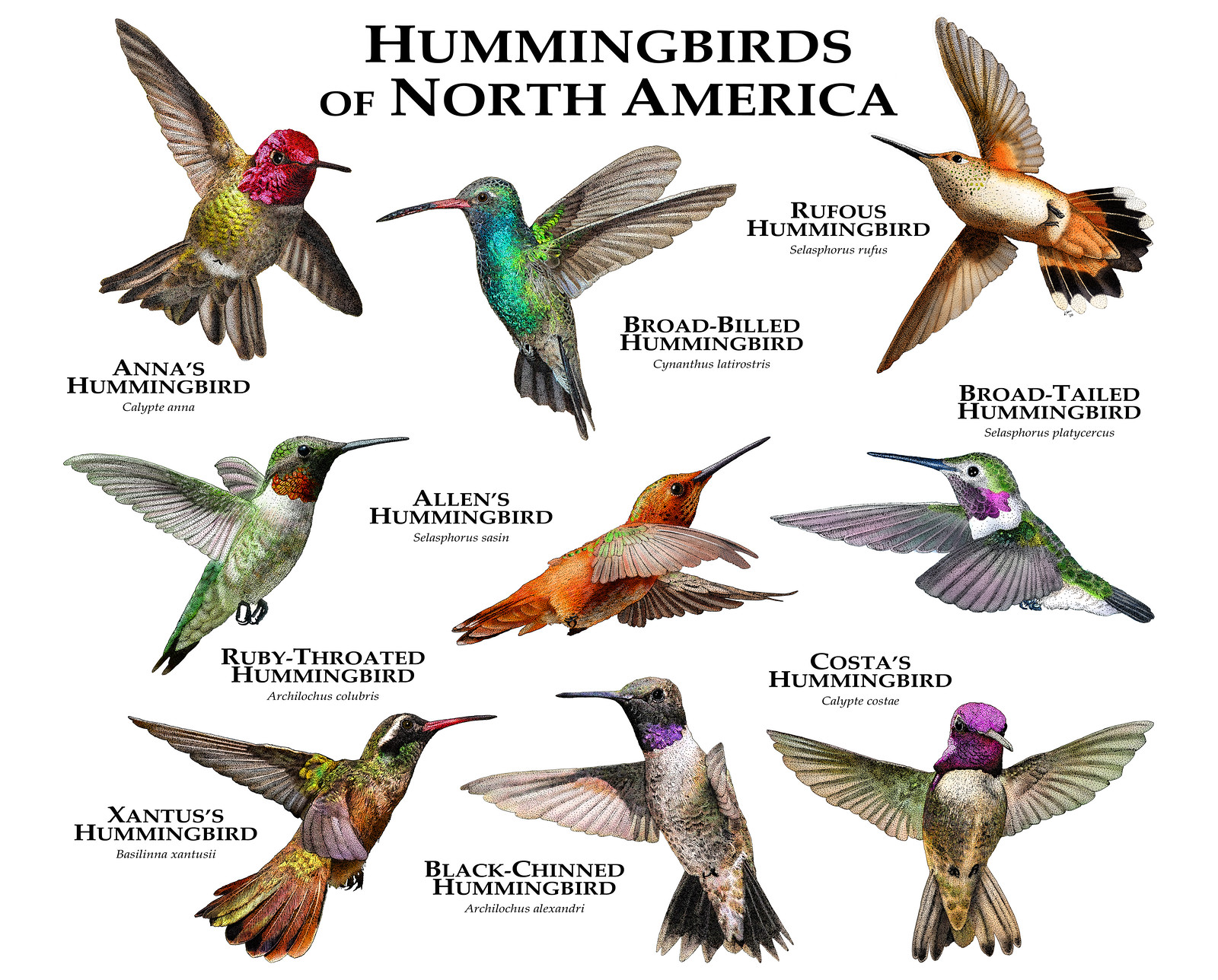This detailed illustration, titled "Hummingbirds of North America" in bold black font at the top, showcases nine vibrant and meticulously drawn hummingbirds, each labeled with their common name and scientific name underneath. Starting from the top left, the Anna's Hummingbird stands out with its pink head, long beak, greenish body, and light to dark brown wings and tail. To its right, the Broad-billed Hummingbird features a teal-green body and slightly longer beak, with light brown wings. Next, the Rufous Hummingbird has an orange tail with black tips, a lighter inner body, and light brown wings. The Ruby-throated Hummingbird sports a distinct ruby-colored throat, a light green body, and white and green wings.

On the second row, Alan's Hummingbird is entirely orange with lighter brown wings and a long beak. Next to it, the Broad-tailed Hummingbird has light purple wings, a green back, and a purple neck. The bottom row includes the Black-chinned Hummingbird with a black head, purple neck, and black-tipped wings, and the Costa's Hummingbird, which has a lighter green body and a purple head.

Lastly, the Xantus’s Hummingbird, depicted with a multicolored body of purple, yellow, and green hues, concludes the collection. Each bird is showcased in rich, diverse colors including shades of red, peacock blue, and various greens, truly highlighting the unique beauty of North American hummingbirds.